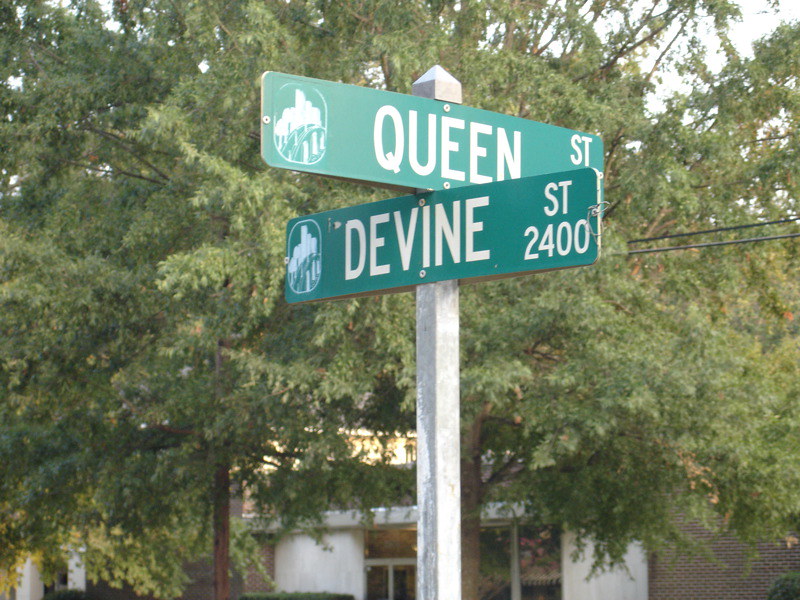In this detailed photograph, the focus is on two intersecting street signs mounted on a white decorative pole. The top street sign, in green with white capital letters, reads "QUEEN STREET." Directly below it, also in green with white text, is "DIVINE STREET," accompanied by the number "2400" in the bottom right corner of the sign. Each sign features a small icon on the left side, appearing to depict a curved bridge-like structure.

The street signs are set at perpendicular angles to each other, with the lower portion of the Queen Street sign partially obscured by the Divine Street sign. The scene is framed by lush green foliage from large trees with brown branches, dominating the background. Additionally, a white building with glass doors and windows is partly visible behind the trees, along with a red brick building with central windows. Power lines are noticeable running beneath the canopy of the large tree, and the bright, white sky casts reflections on the buildings.